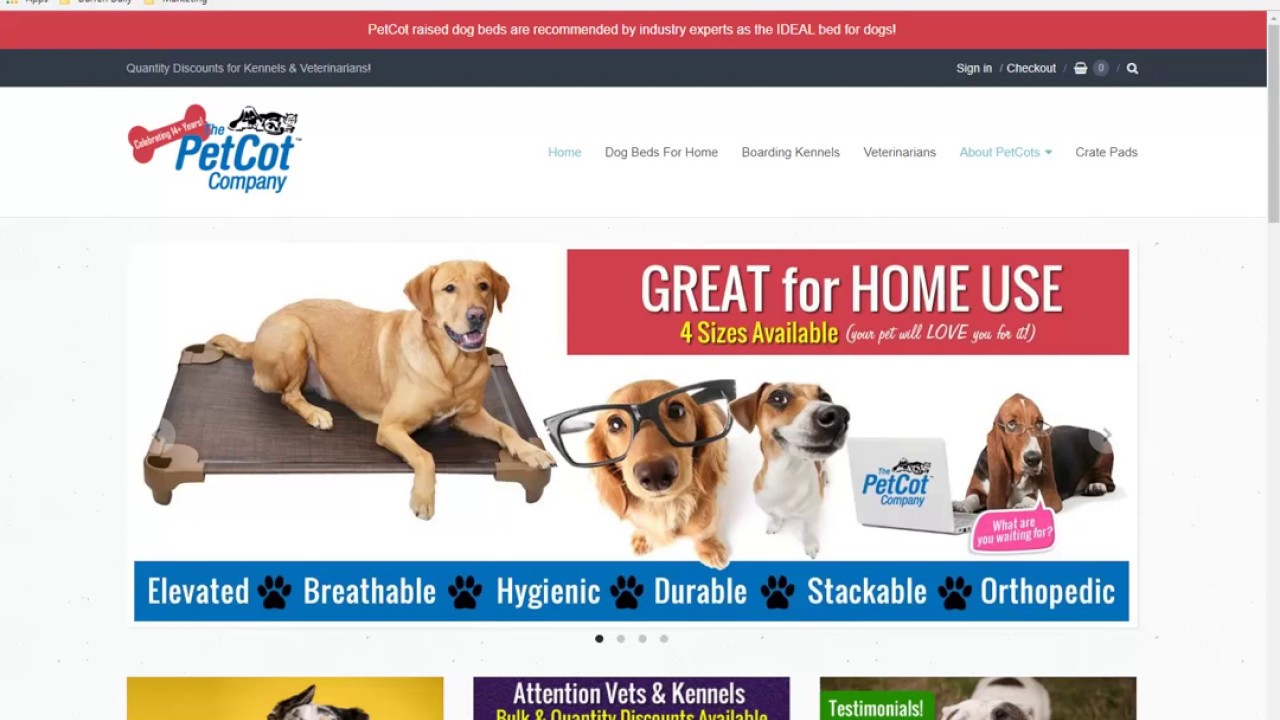The image features a promotional graphic for **Pet Cot raised dog beds**. The top of the image has a **red border** with text that reads, "**Pet Cot raised dog beds are recommended by industry experts as the ideal bed for dogs**." Below this, on a **black background**, the graphic includes the text, "**Quantity discounts for kennels and veterinarians**," accompanied by icons for **sign-in, shopping basket, and a search function**.

The lower portion of the graphic has a **white background** with a red dog bone icon stating, "**Celebrating 16 years**." It also includes the text, "The Pet Cot Company" followed by menu options such as "**Home, Dog Beds, for Home, Boarding Kennels, Veterinarian**, and more." A **short-haired brown dog** is displayed comfortably lying on the raised bed, which is advertised in a **red box** with the caption, "**Great for home use - Four sizes available - Your pet will love you for it**."

Beneath this, there are bullet points highlighting the features: "**Elevated, breathable, hygienic, durable, stackable, orthopedic**." An additional note reads, "**Attention vets and kennels: Bulk and quantity discounts available**."